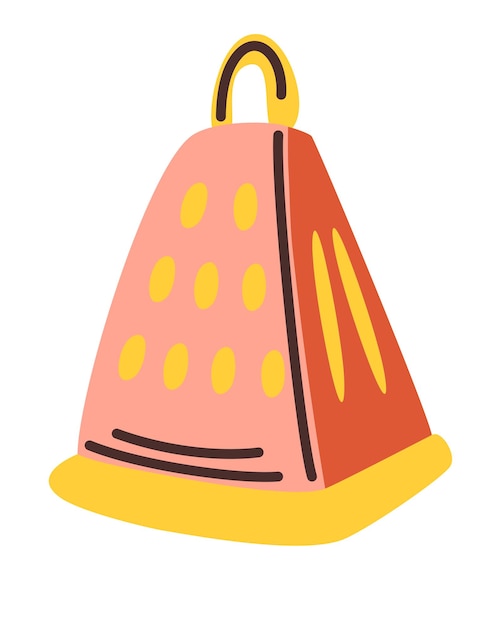This image is a stylized, cartoon-like vector illustration of a cheese grater. The grater features vibrant, non-traditional colors: the front facing side is a pale pink with yellow grating holes arranged in rows of two, three, and four. The left side is a bright orangey-red, showcasing long, vertical grating slots. The handle is yellow with a black stripe down its center, and the base is a thick, curved yellow section. There are additional black lines adding detail to the bottom and edges of the grater. The entire illustration is set against a stark white background, emphasizing its playful, animated design.